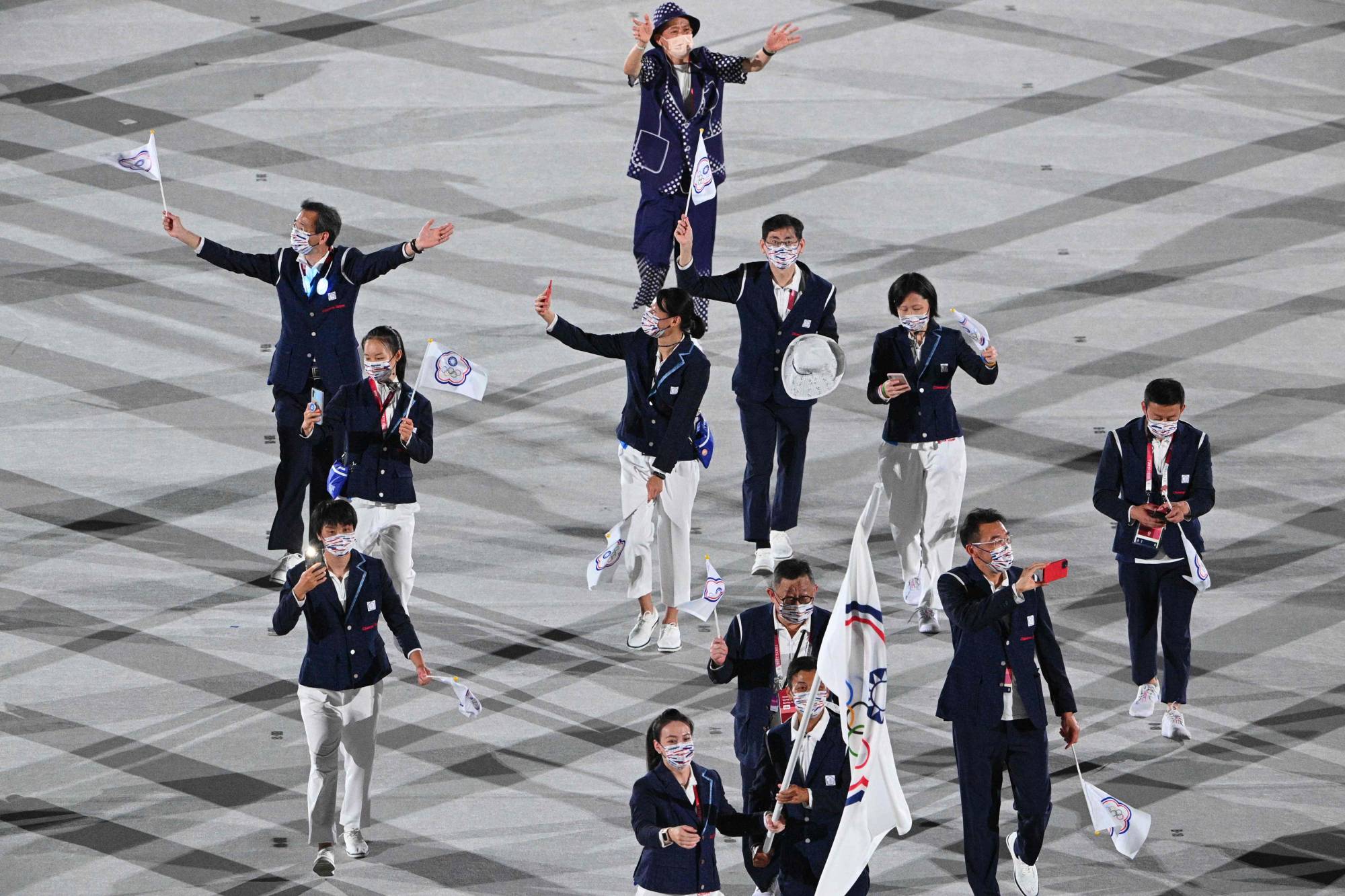The image depicts a cheerful group of young Asian men and women, likely from the South Korean Olympic team, participating in a parade during the COVID-19 pandemic, as evidenced by their white face masks. They are attired in a distinct uniform: women in white pants, blue jackets, and white tennis shoes, and men in blue pants, dark tops with white shirts underneath, button-down jackets with four buttons, and white tennis shoes. They are walking on a gray and white patterned floor, possibly in an Olympic stadium, creating noticeable shadows. The group is waving flags enthusiastically; most hold small national flags, while a prominent male figure at the front carries a large flag featuring the five Olympic rings. The scene is vibrant and animated, with some participants taking pictures on their phones, further highlighting their excitement and contentment.